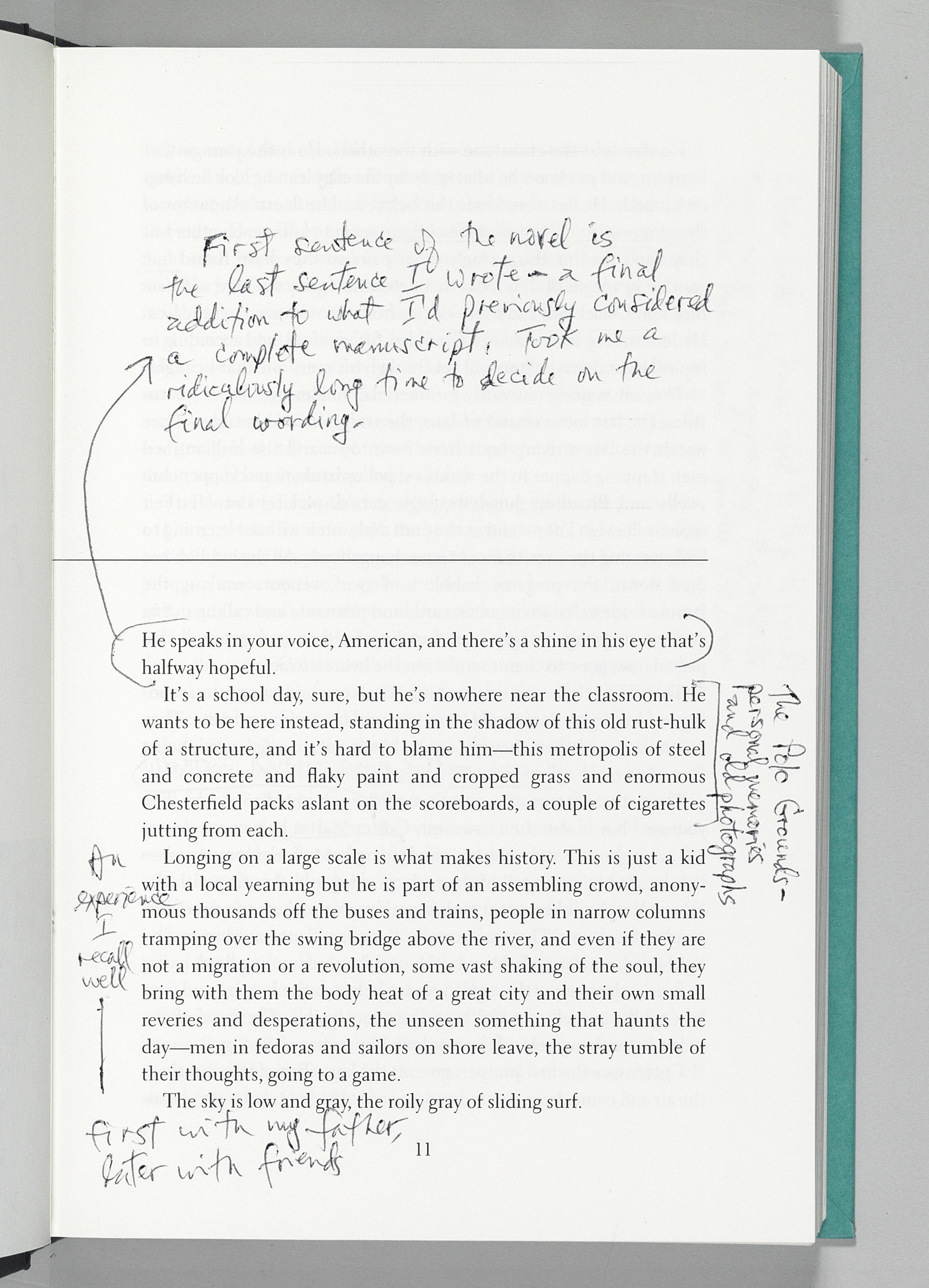The image is a photograph taken from above, showcasing an open hardcover book lying flat on a light gray, stenciled background. The primary focus is on the right-hand page of the book, which is turned to page 11, as indicated by the number at the bottom center of the page. The top half of the page features a handwritten note stating, "The first sentence of the novel is the last sentence I wrote. Final addition to what I previously considered the complete manuscript took me a ridiculously long time to decide on the final word." This note connects via an arrow to a paragraph in the otherwise blank top half of the page. Beneath this, the lower half of the page contains printed paragraphs of text. Additional handwritten notes are visible in the margins: one written vertically along the right side, and more notes scribbled in the middle left and bottom left margins. The blue hue of the book's back cover peeks through on the far left side of the image.